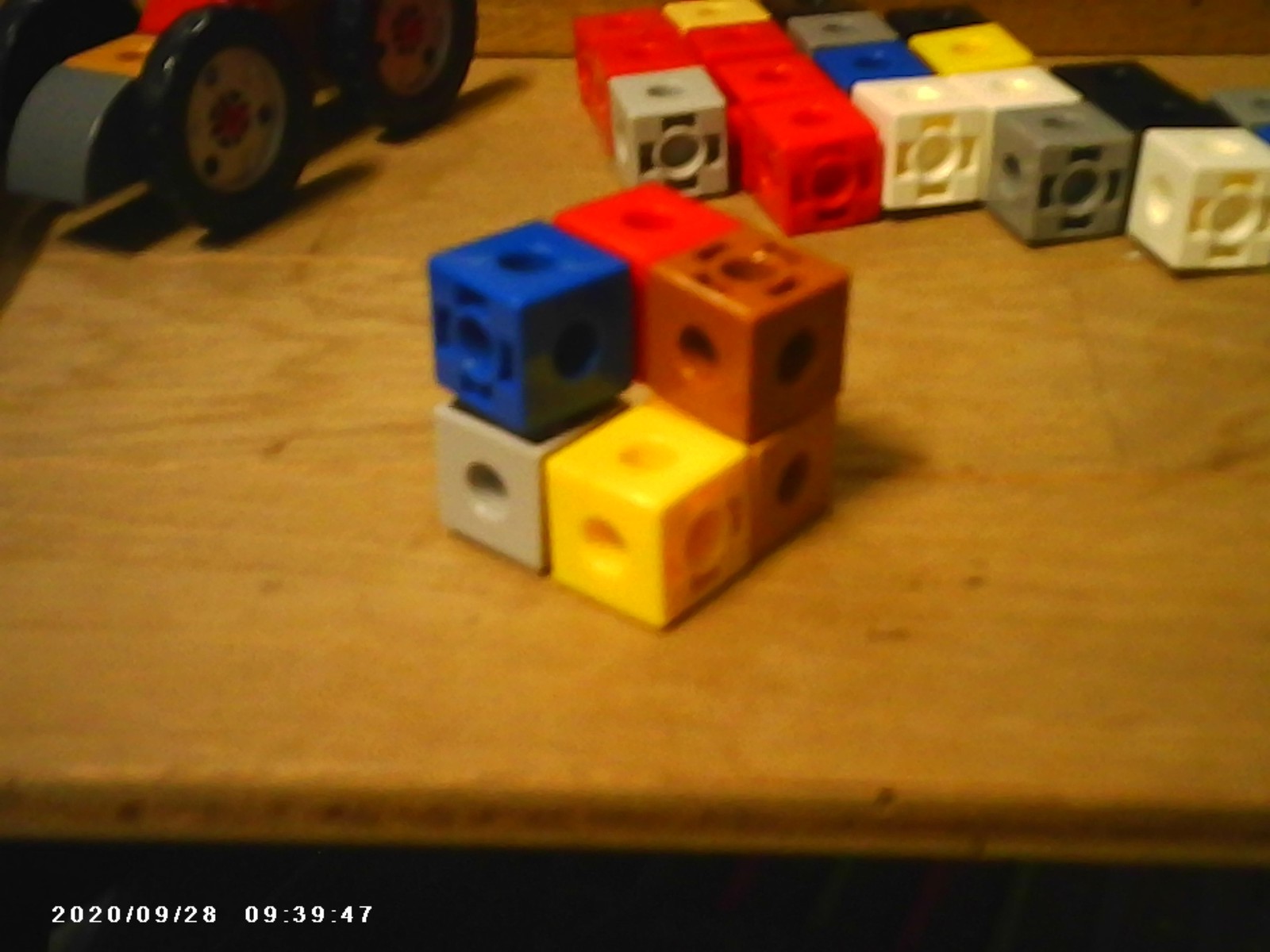The image depicts a slightly out-of-focus, color photograph taken on September 28, 2020, at 9:39:47 AM, as indicated by a white time and date stamp in the bottom left corner. The scene is set on a well-used, light-colored wooden tabletop, bearing some stains. On the upper left, there's a children's toy made from building blocks, partially visible with two large, black-and-gray tractor wheels. The toy includes a rounded front piece and some yellow and red blocks, casting a shadow on the table.

In the foreground, a stack of seven small, cube-shaped building blocks is arranged in a 4-3 configuration, forming a 'V' shape on the top tier and a square on the bottom. The top row consists of blue, red, and brown cubes, while the bottom row has gray, yellow, tan, and another block obscured at the back. These blocks have ring-shaped protrusions for interlocking, unlike typical solid Lego studs.

In the background, there are five visible rows of additional blocks lying flat. These are organized in a sequence including red, gray, yellow, black, blue, and white blocks, with more extending out of the frame to the right. The blocks appear to be around half an inch to an inch in size.